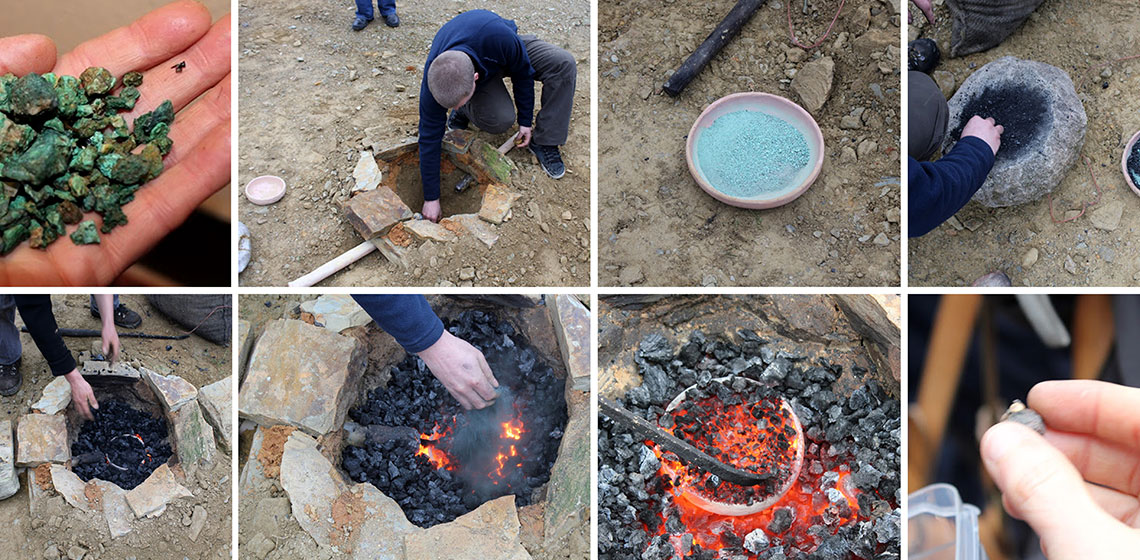The image collage consists of eight photographs neatly arranged with distinct white spaces separating them; one horizontal white line and three vertical white lines create a grid-like structure. 

- The top-left photograph shows a person's palm holding a collection of green rocks, possibly artifacts or minerals.
- To its right, a man dressed in a blue shirt and gray pants is depicted excavating a hole, hinting at an archaeological dig.
- The third image features a beige-colored bowl filled with a light blue-gray, sandy substance, indicative of a sample or material analysis.
- The fourth photo captures a sizable rock displaying a black substance, perhaps charcoal or a mineral deposit.
- In the bottom row, the first picture on the left presents a circular arrangement of rocks, resembling a constructed formation or a symbolic structure.
- The subsequent image shows the same dark substance from the previous rocks, now glowing, suggesting it is being heated.
- The second-to-last photo continues this sequence, displaying the material glowing even more intensely, indicating a high-temperature process.
- The final image features a hand holding a small, black pebble, likely a sample collected from the site.

This detailed collage visually narrates the steps of an archaeological investigation, from excavation to material analysis and processing.